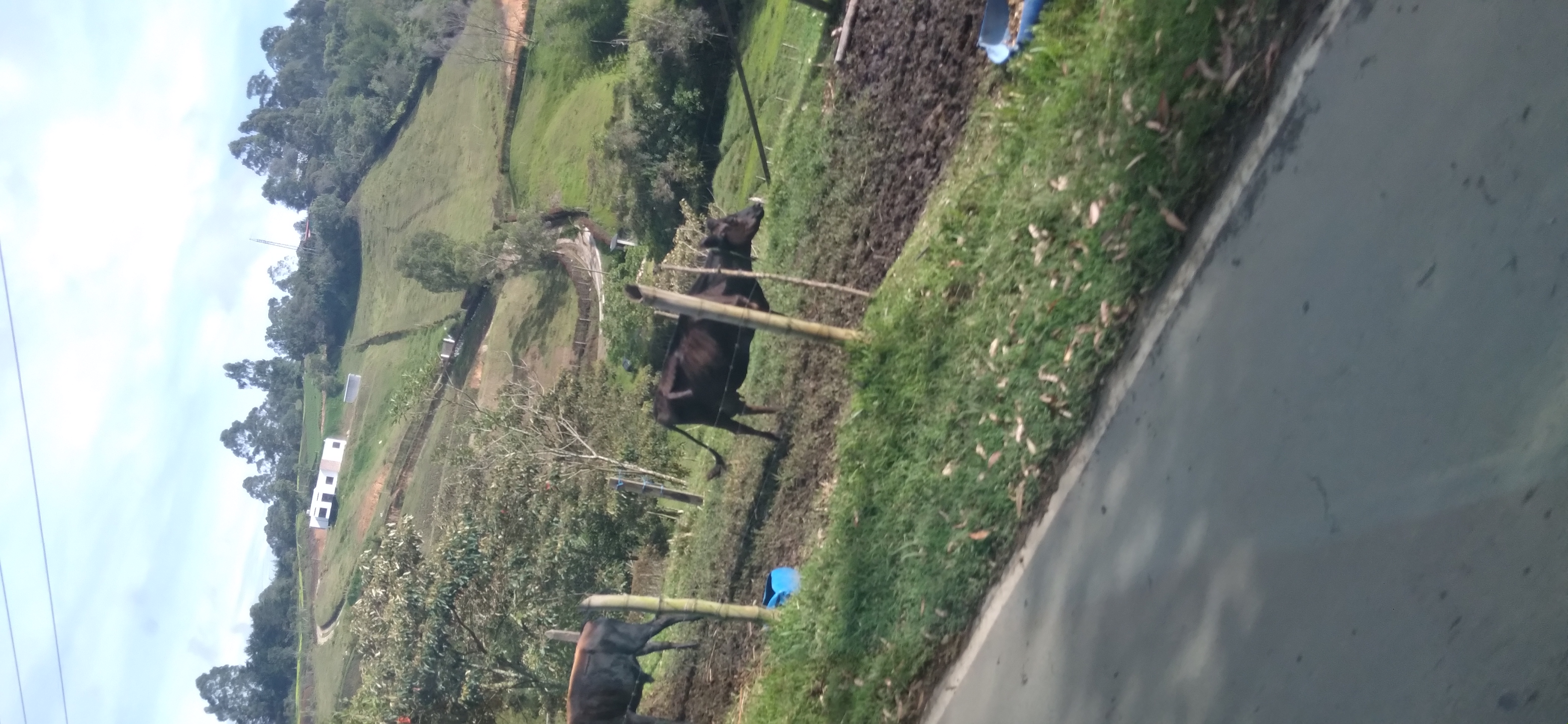This vertical color photograph captures a picturesque countryside scene on a sunny but slightly cloudy day. The photo is taken from the road, looking over a bamboo fence that separates the photographer from a pasture. In the foreground, a large dark brown, almost black cow with horns stands prominently, appearing to be the focal point of the image. Nearby, there are blue containers, likely holding food for the animals. Just behind the main cow, another large animal is partially visible, showing only its back half—it could be another cow, a horse, or a donkey. The pasture around them is tilled, with dark soil ready for planting, surrounded by vibrant green grass. The scene stretches out to reveal a hill in the distance, blanketed with trees and leading up to a white house perched at the top. To the left, a black concrete sidewalk edged with fallen leaves meanders through the lush landscape, adding to the serene and idyllic atmosphere of the countryside location.